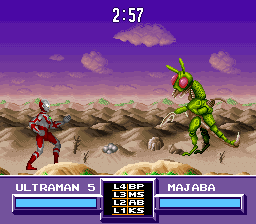This image is likely a screenshot from a retro-style video game, characterized by its pixelated graphics that evoke a sense of nostalgia for older gaming aesthetics. The scene appears to be set in a fighting game, evident from the combat-oriented elements and character positioning. The background showcases a desert landscape under a vivid purple sky, a stark and surreal setting for a battle. 

On the left side of the screen stands a red and silver robot named "Ultraman 5," as indicated by the label above its health meter, which is displayed in blue. This mechanical combatant seems ready for action. On the right side, there is a giant green praying mantis-like creature called "Machaba," distinguishable by its bright red eyes and a formidable tail. Both characters are poised for combat, suggesting an impending clash.

The detailed health meters below the characters add to the classic fighting game feel, indicating each character's remaining vitality and enhancing the competitive atmosphere of the scene. The juxtaposition of the robot and the alien insectoid in a desert setting under a purple sky creates a unique and imaginative visual experience reminiscent of vintage video gaming.